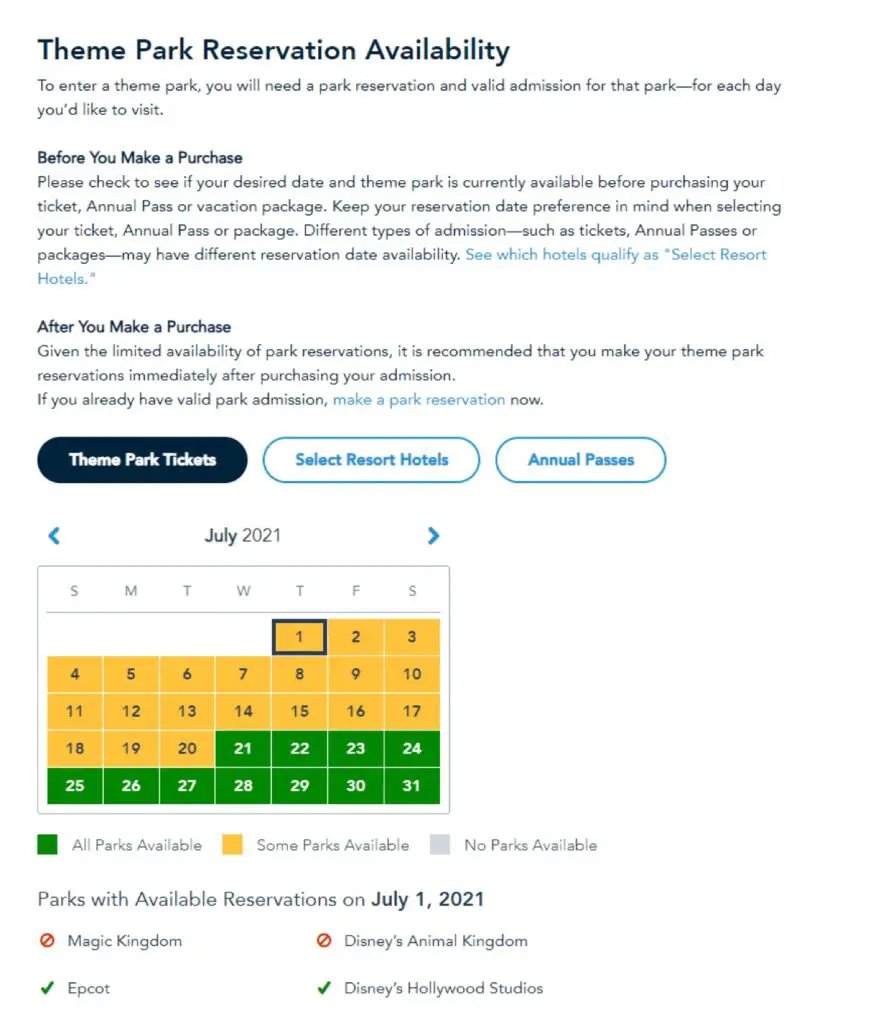The screenshot depicts a section of Disney's website showcasing theme park reservation details. At the very top, in bold black font, is the headline: "Theme Park Reservation Availability." Beneath this, there's a notification: "To enter a theme park, you need a park reservation and valid admission for that park for each day you'd like to visit." 

A secondary headline follows: "Before You Make a Purchase," accompanied by a paragraph, and then "After You Make a Purchase," followed by another paragraph. Below this information, three rectangular buttons with rounded corners are displayed. The first rectangle says "Theme Park Tickets" in white font on a black background. The second rectangle, outlined in blue, contains "Select Resort Hotels" in blue font. The third rectangle, similarly outlined in blue, reads "Annual Passes" in blue font.

Below these options, a calendar is visible, labeled at the top as "July 2021." The calendar shows the entire month, with dates from July 1st to 20th highlighted in gold, indicating some parks are available. Dates from July 21st to 31st are highlighted in green, denoting all parks are available. Grey, which isn’t represented in this snapshot, would indicate no parks are available.

At the very bottom, a line delineates parks with available reservations on July 1st, 2021, listing Magic Kingdom, Epcot, Disney's Animal Kingdom, and Disney's Hollywood Studios.